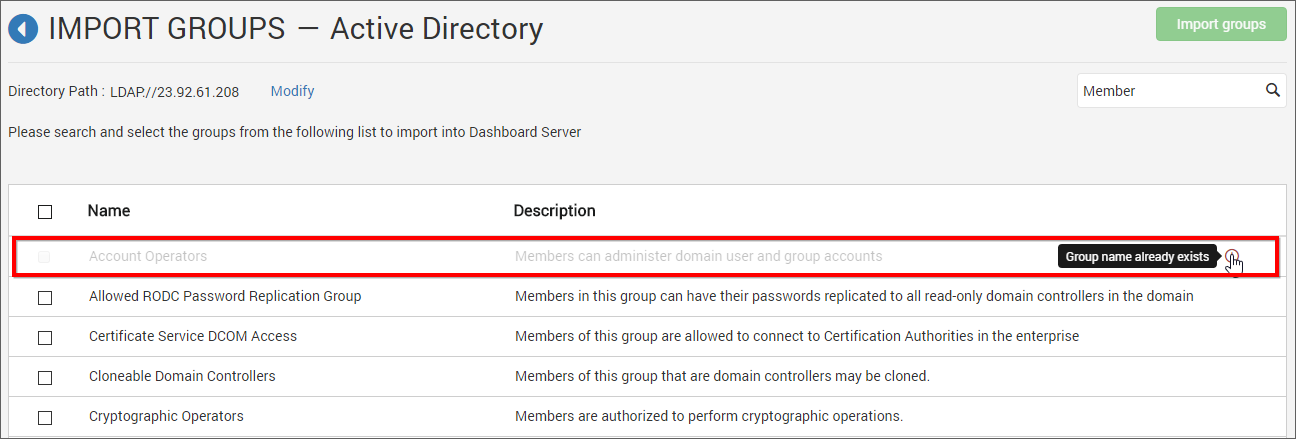The webpage displayed is for importing groups from Active Directory. At the top of the page, there's a heading that reads "Import Groups" with a back arrow in front of it, followed by "Active Directory" on the same line. A green button labeled "Import Groups" is also present on this line.

Just below this, the page features a section labeled "Directory Path" with a value of "LDAP\2392-61-208" and a "Modify" button next to it. Opposite to this is a "Member" search box, which includes a magnifying glass icon.

Further down, the instructions indicate: "Please search and select the groups from the following list to import into Dashboard Server." 

A white rectangular checklist spans the width of the page. The checklist header reads "Name and Description." The first entry is highlighted in red and labeled "Account Operators," with a description stating "Members can administer domain user groups in account," followed by a note: "Group Name already exists." 

Subsequent checklist entries include:
- **Allowed RODC Password Replication**: A tick mark indicates selection, with the description "Members of this group can have their passwords replicated to all read-only domain controllers in this domain."
- **Certificate Service DCOM Access**: Features a checkbox with the description "Members of this group are allowed to connect to certification authorities in the enterprise."
- **Clonable Domain Controllers**: This checkbox indicates that "Members of this group that are domain controllers may be cloned."
- **Cryptographic Operations**: The final checkbox states "Members are allowed to perform cryptographic operations."

The page facilitates the selection of specific Active Directory groups for importation, accompanied by descriptive details for informed choices.